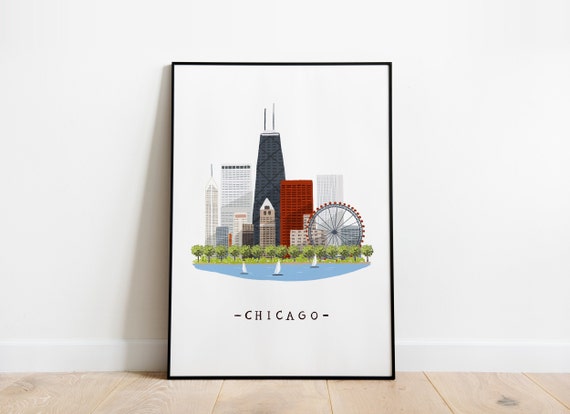The image captures a framed print of an illustrated depiction of downtown Chicago, positioned atop a light, ashy wood table and leaning against a pristine white wall with white baseboards. The thin black frame outlines a white background where the word "Chicago" is written at the bottom. The artwork features a cartoon-like animation of the city's skyline, including a very tall gray building resembling the Sears Tower with radio antennas on top, a distinctive red building, and several other silver-gray skyscrapers. In the foreground, there's a serene lake with three sailboats with white sails, bordered by a lush green tree line. Further in the distance, a Ferris wheel turns, adding a nostalgic touch to the vibrant cityscape. The room's lighting creates a soft shadow behind the framed print, enhancing its presence in the space.